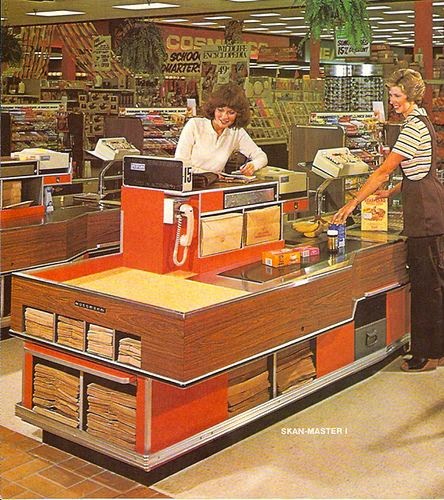This detailed photograph appears to transport viewers back to a grocery store scene from the late 1960s or 1970s. Central to the image is a cash register area marked with the number 15 in black lettering, featuring an orange body complemented by natural-looking wooden paneling. The cash register’s conveyor belt displays various grocery items, including bananas, an orange box, a pink box, what appears to be a yellowish box of cereal, and a jar of instant coffee.

To the right of the register, slightly near the top right, stands a smiling white woman with short, neck-length blonde hair that is teased back. She is dressed in a distinctive striped polo shirt with white, green, and lighter green stripes, paired with a brown smock, brown pants, and brown-red shoes. This woman is presumably the cashier, diligently scanning items using a scanner positioned on the right side of the register, and directing them down towards the end part of the table where several paper bags are kept.

In front of her is a second woman — the customer — visible only from the waist up. She has brunette, poofy shoulder-length hair and is wearing a white Henley shirt. This woman appears to be engrossed in an activity, possibly looking at a magazine, as her brown wallet rests on the register platform. In the background, multiple aisles are discernible but not detailed, showcasing the expansive layout of the store. Hanging plants add a touch of decor above each register, while rows of sunglasses are faintly visible, hinting at the various sections of the supermarket, which also includes cosmetics and school supplies. The store's ambience, marked by bright orange, brown, and yellow hues, emphasizes the nostalgic feel of the era. A watermark at the bottom, "ScanMaster 1," suggests that this image has been digitally archived.